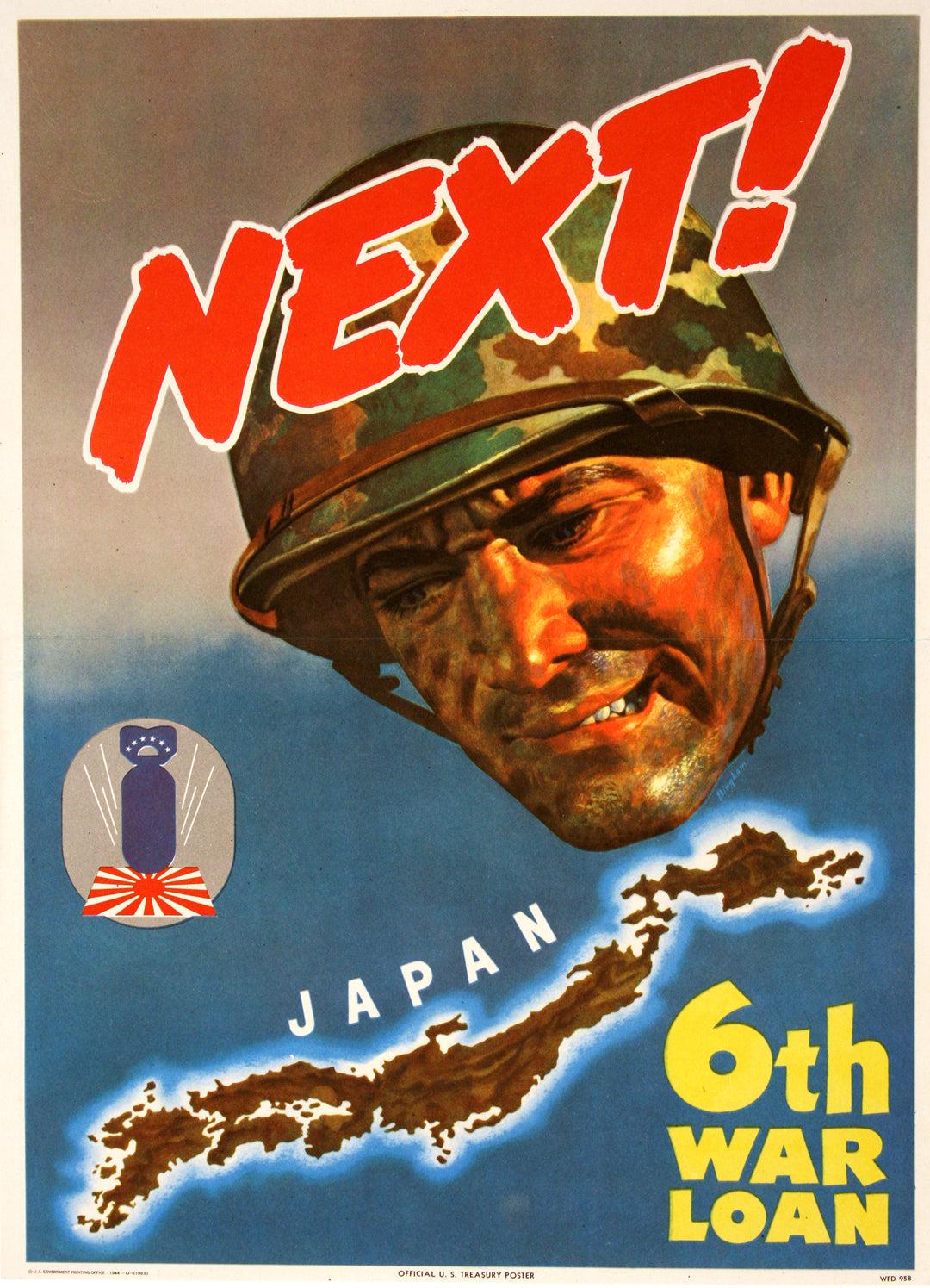This vintage military poster features a vertical rectangular layout typical of 1950s or 1960s design. Across the top, the word "NEXT!" is boldly displayed in large red letters with a white border, written diagonally over the helmet of a soldier who appears grim and focused. The soldier is wearing a camouflage pith helmet and gazes toward an illustration of Japan, which is marked in brown and labeled "Japan," showing all its islands. Beneath the soldier's head, the text “SIXTH WAR LOAN” stands out in substantial yellow letters, emphasizing a call to action. On the left side of the poster, there is a striking depiction of a blue bomb with a blue handle, seemingly falling onto the red circle of the Japanese rising sun flag with rays emanating outwards, reflecting a message of wartime aggression. At the very bottom, the insignia "Official U.S. Treasury Poster" confirms its purpose as wartime propaganda, likely intended to encourage financial support for World War II efforts.